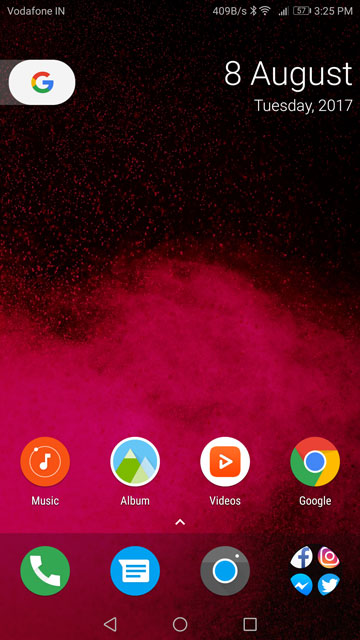In the upper left-hand corner of the phone screen, the text "Vodafone IN" is displayed, with "Vodafone" spelled as V-O-D-A-F-O-N-E and "IN" in capital letters. On the upper right-hand corner, it shows the reference "4098/S." Adjacent to these, there are icons for Bluetooth, Wi-Fi, and cellular signal. The battery level is indicated at 57%, and the time shown is 3:25 p.m. 

Beneath the "Vodafone IN" text, there's a white oval containing the letter "G," representing the Google app. On the right side, the date is displayed as "8 August, Tuesday, 2017."

The phone's background features a red mist or fog with splatter-like patterns. There are four primary apps displayed on the main screen, organized from left to right: Music, Album, Videos, and Google. 

At the bottom of the screen, in the docked section, there are four more apps bookmarked. From left to right, these include the Phone app (with a green icon), the Messaging app (with a blue icon), a third app represented by a blue circle, and a folder containing four social media apps: Facebook, Instagram, Messenger, and Twitter.